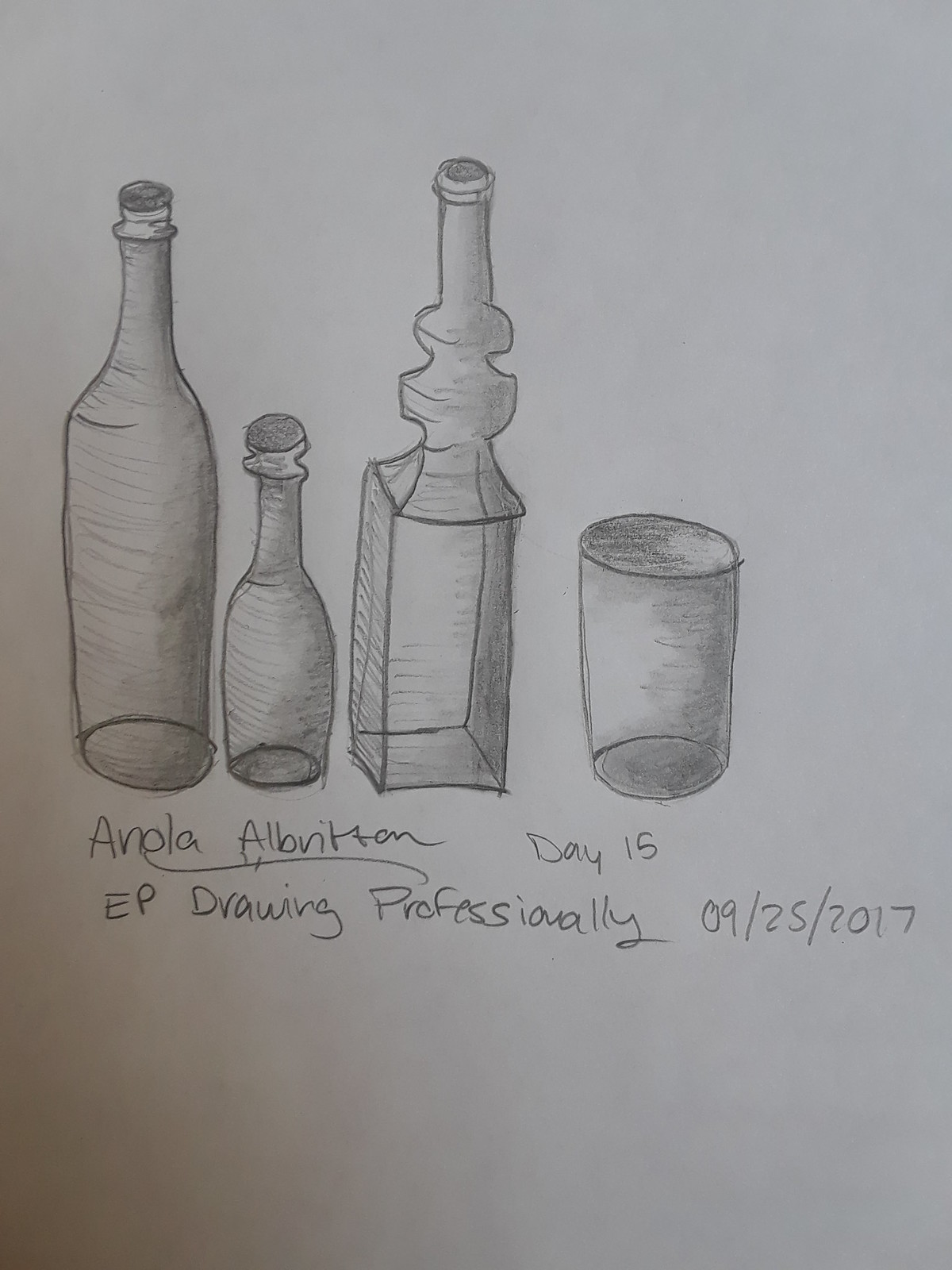This detailed pencil drawing on white paper depicts three distinctive bottles and a drinking glass. The bottle on the left resembles a wine bottle and has a cork. The center bottle is smaller with a long, thin neck and also features a cork. The third bottle on the right, distinguished by its square base, notched long neck, and cork, stands next to a smooth, cylindrical drinking glass. Written at the bottom of the drawing in pencil are the words "Enola, Albritton, Day 15," underlined, followed by "E.P. Drawing Professionally, 05-25-2017."